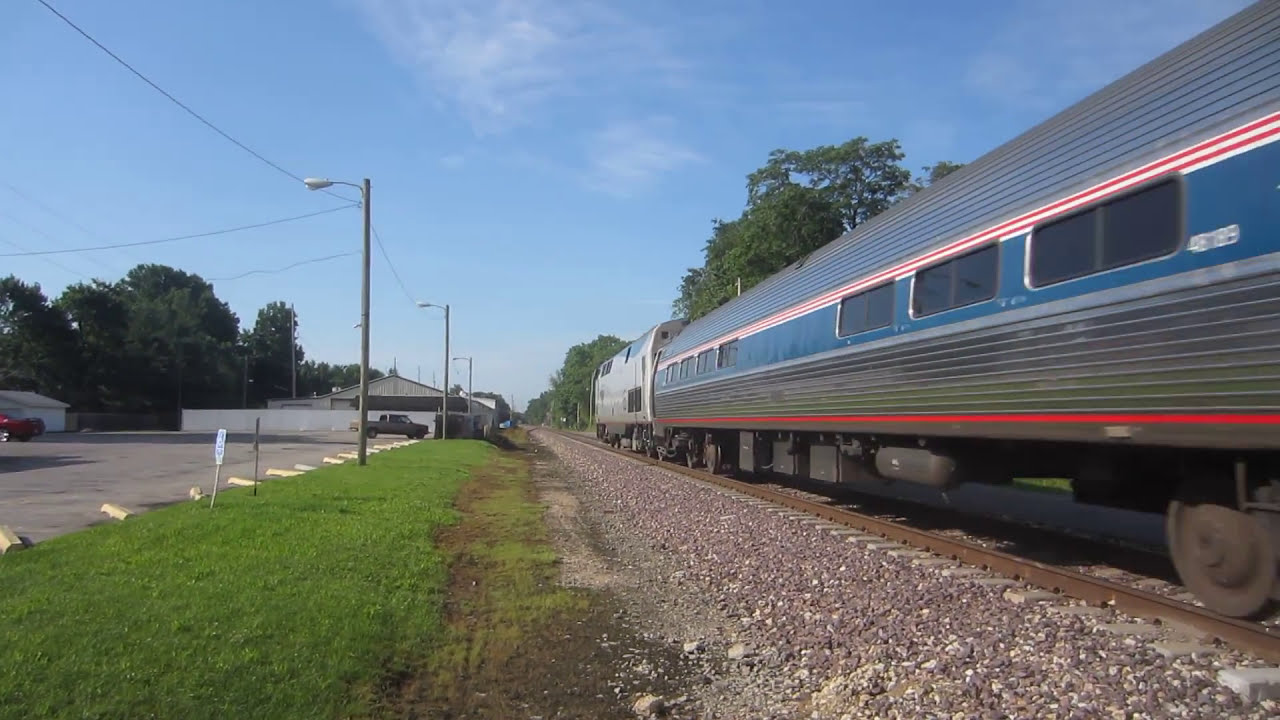In the photorealistic image, the right side prominently features a sleek gray train with large blue, red, and white stripes running along its side. The train extends from the right edge towards the center, progressing into the distance along straight, rusted tracks that are supported by brown gravel. The train's side is adorned with several rectangular windows. The backdrop of the image behind the train consists of a clear blue sky dotted with some white clouds, and is framed by green leafy trees peaking over the train.

On the left side of the image, a patchwork of grass and dirt transitions into a slate gray parking lot marked with yellow indicators. The parking lot houses a brown pickup truck and a red car. Further in the distance, one can see small and large white buildings amidst scattered green trees. Several light posts, equipped with brown power lines and large street lamps, line the parking lot. The entire scene is set under a bright, clear sky, adding to the vivid realism of the photograph.